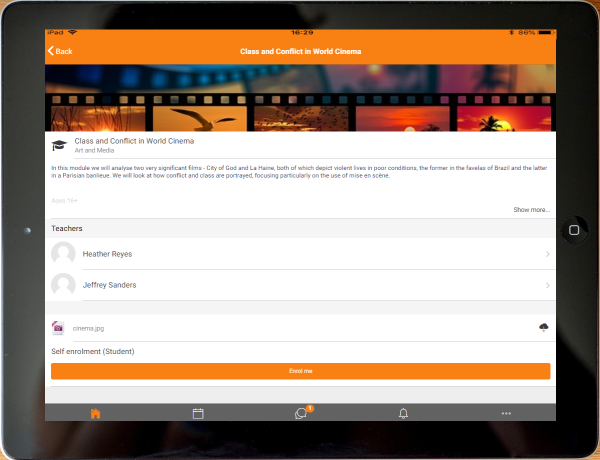A detailed image caption could be formulated as:

"Displayed on an iPad screen, the website features a prominent orange banner at the top, adorned in the center with white text reading 'Class and Conflict in World Cinema.' Below the banner, an image of film strips suffused with red and orange tones depicts sunrises and birds in flight, imparting a warm, vibrant atmosphere. Dominating the lower two-thirds of the page is a large white rectangle. At the top-left corner of this rectangle sits a small graduation cap icon, next to which the course title 'Class and Conflict in World Cinema' is displayed in dark gray font. Beneath this title, the subtitle 'Art and Media' is written, followed by course details including a list of instructors. The page offers an opportunity for students to enroll, indicated by the phrase 'self-enrollment (student)' in smaller text."